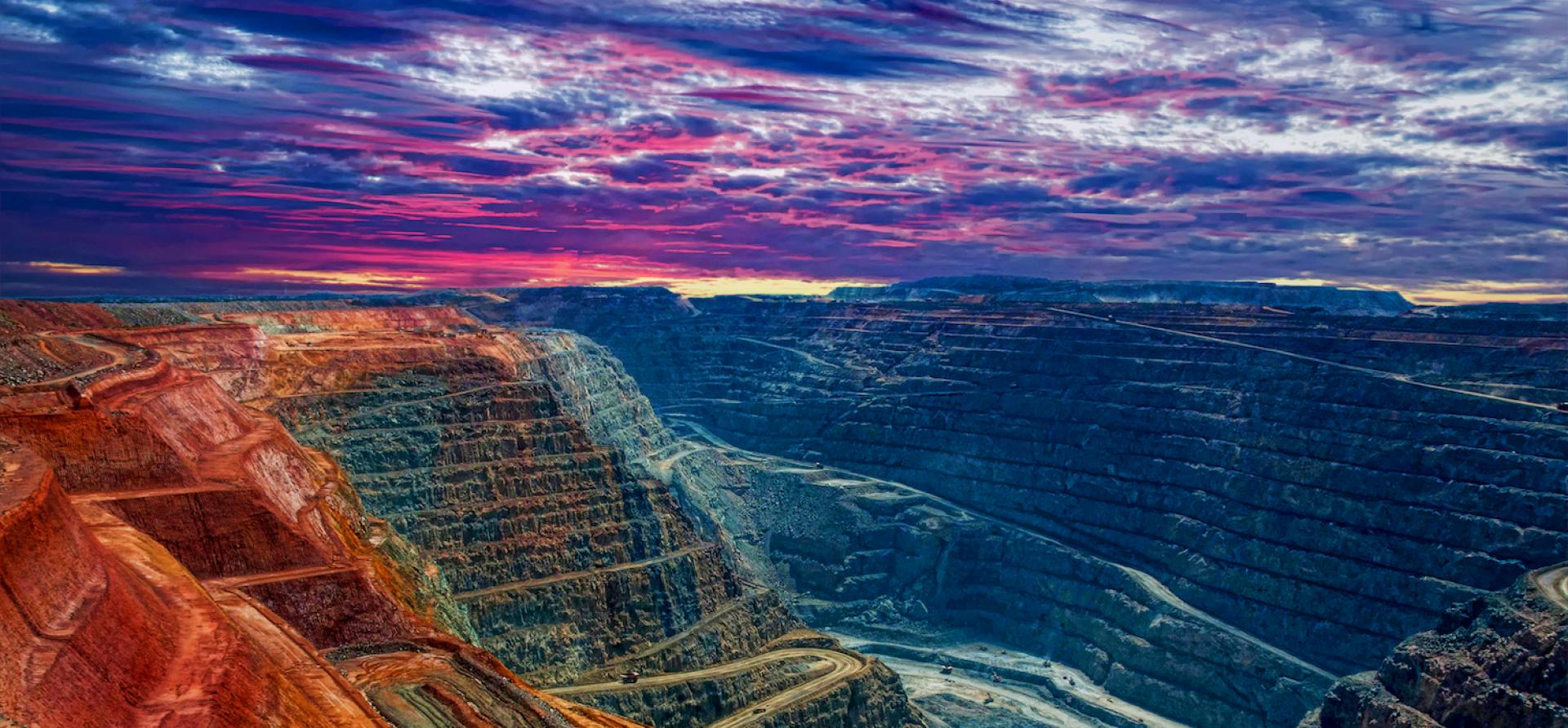A horizontally aligned rectangular photograph captures the breathtaking expanse of the Grand Canyon at sunset. The image reveals a vivid and intricate canyon landscape with the Colorado River winding at the basin. The right side of the river is cast in deep shadows, highlighting the dark, almost black cliffs due to the lack of light. In contrast, the left side features cliffs brightly illuminated, showcasing layers of greenish-brown and striking orange hues at the top.

The brilliant sky above is a spectacle of its own, filled with feathery white clouds mixed with shades of pink, dark blue, and hints of gray, creating a dramatic and colorful atmosphere. The terraced rock formations ascending the canyon walls on the left are adorned with shades of blue, orange, and red, providing a picturesque view of the naturally sculpted landscape. The middle left area reveals what appears to be a roadway perched atop a rocky outcrop, adding a touch of human presence to the vast wilderness. The horizon line marks the transition from light-colored sky at the bottom to vibrant blue and purple tones, interspersed with patches of white and lilac, mirroring the vibrant colors found throughout the canyon. The interplay of light and shadow, combined with the rich, varied colors of the rocks and sky, creates a detailed and mesmerizing depiction of this natural wonder.